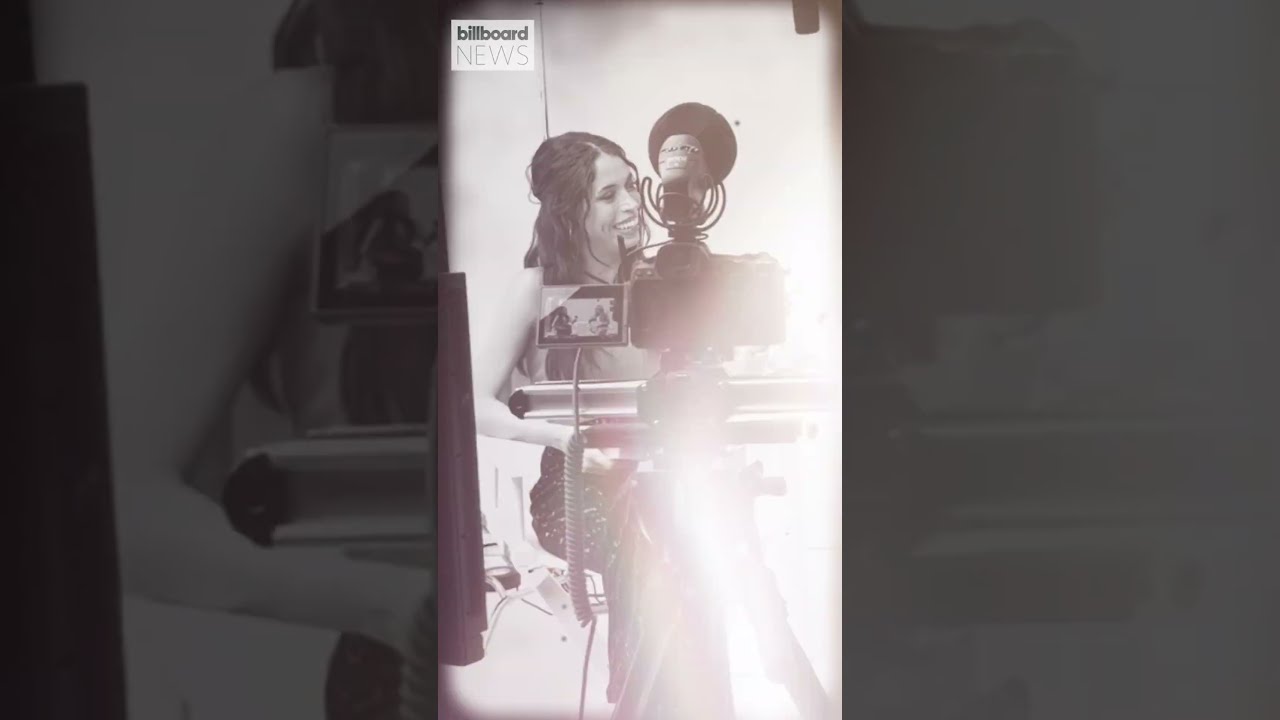The image is a horizontal, rectangular photograph predominantly in black and white, with grayed-out areas on both sides. In the center is a narrower white rectangle featuring the main subject: a woman with long dark hair, smiling and looking to the right. She is seated in a light-colored chair with metal legs and is wearing a sleeveless black dress. A close-up of her location on the grayed-out left side suggests she is positioned in front of a window, though it's mostly obscured by glare. The woman appears to be involved in a photoshoot or video recording session, as indicated by the presence of a video camera in the foreground. The camera, equipped with a flashbulb on top and a microphone, is filming the woman, and its display screen can be seen capturing her image. Additionally, another figure, possibly a superimposed or cartoon character, appears next to or in front of her, adding a layer of visual complexity. The top-left corner of the photograph displays the words "Billboard News" in distinct fonts within a white square, further contextualizing the scene.